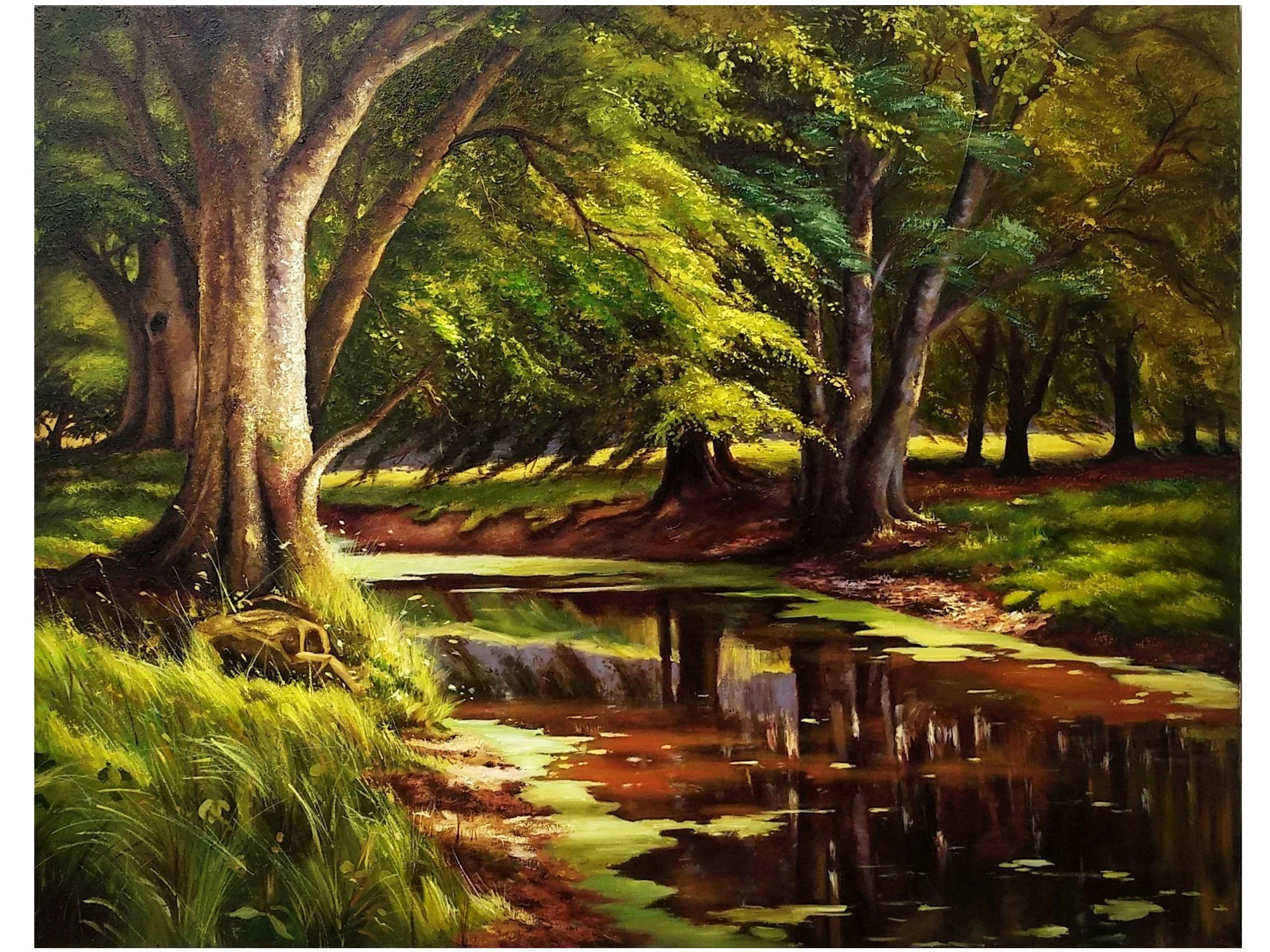This captivating illustration presents a serene, untamed landscape featuring a slow-moving, muddy brown river or creek at its center. Lining the waterway are lush, verdant trees, some displaying darker green leaves while others showcase lighter, almost amber and yellow-tinted foliage, suggestive of either spring or summer. The water is flanked by green patches, likely rich in algae or moss, contributing to the scene's natural charm. On the right side of the picture, a dirt path weaves gently into the distance, enhancing the sense of tranquility. Meanwhile, the foreground boasts high tufts of grass, with varying hues that hint at the presence of insects, offering a snapshot of a thriving ecosystem. The overall atmosphere is one of peacefulness and untouched beauty.